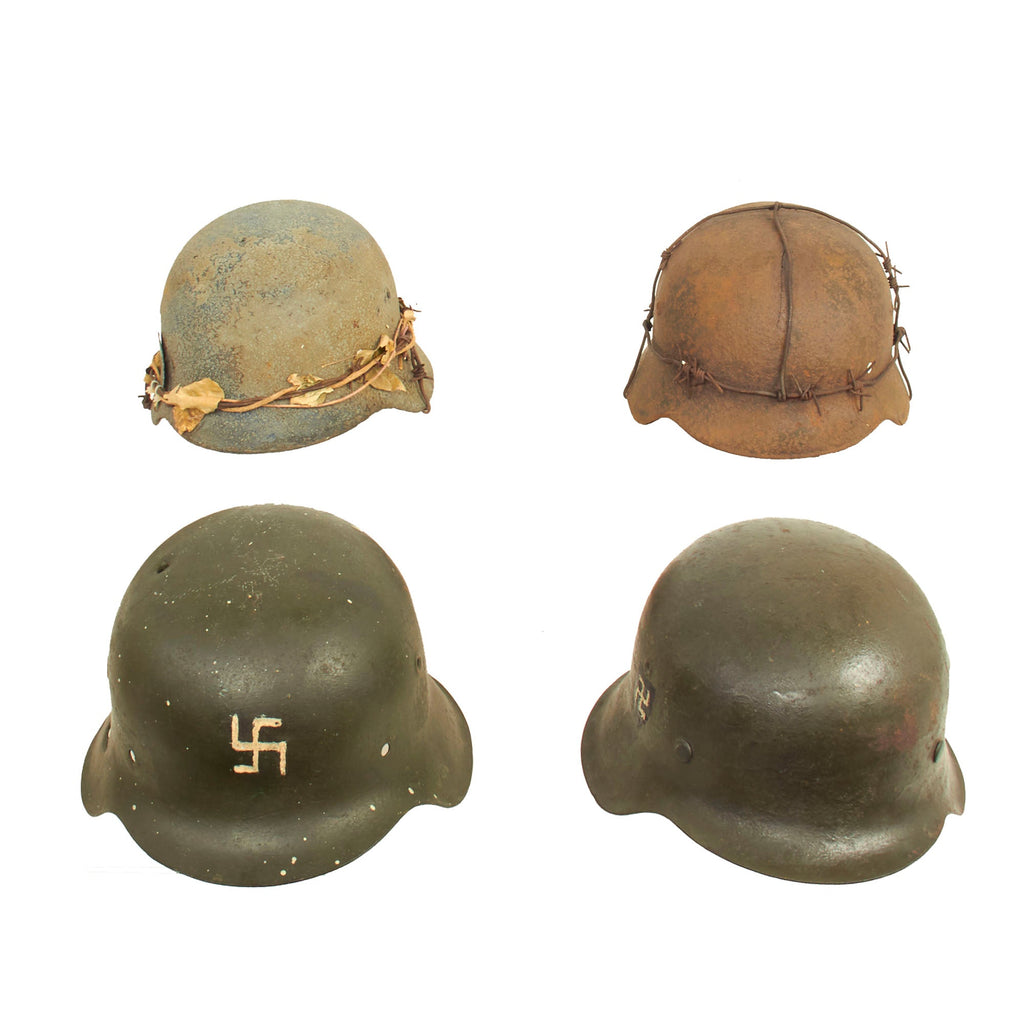This photograph depicts four distinct World War II-era helmets, each revealing a rich tapestry of history through their worn exteriors. Arranged in two rows of two, the lower pair exhibit more intricate details, while the upper two are adorned with additional elements. The lower left and right helmets are characterized by their notable white swastikas; the left one bearing the symbol on its front and the right on its side. Both helmets, showing signs of extensive wear, have a dark, faded hue of blackish-brown.

In contrast, the two helmets at the top showcase a different kind of wear, with one featuring a light greenish-blue base, as if it's been exposed to elements or buried in dirt. The helmet on the upper right is predominantly brown, accented with barbed wire that wraps around its front and over the top, displaying rust and age. The upper left helmet has a more natural aesthetic, encircled by what appears to be tree branches or vines. All four helmets share the classic WWII design with flaps extending over the ears, but the bottom pair appears more robust and substantial in comparison. This juxtaposition of helmets not only highlights the passage of time but also the diverse environments and battles they have likely witnessed.